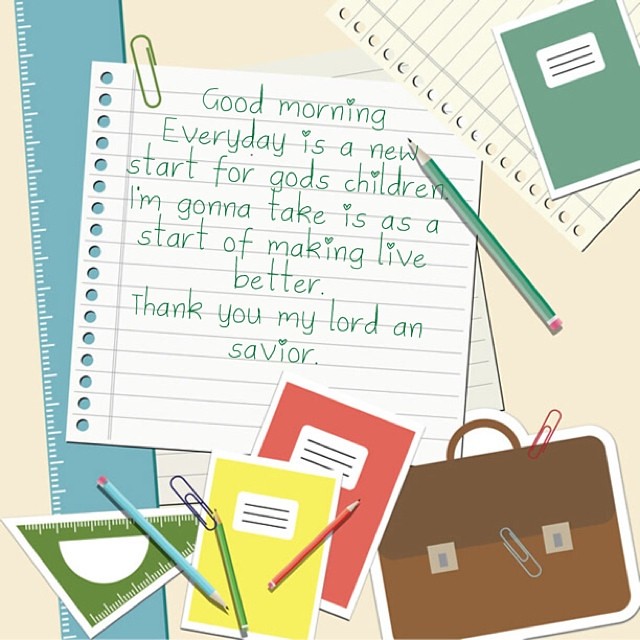The image is a computer-generated piece of graphic art with a beige background. On the left-hand side, a blue ruler runs vertically alongside a red protractor positioned at the bottom. Scattered around are various school supplies, including a red and yellow notebook, paperclips, and several pencils—two green, one red, and one blue. A miniature blue book bag is also present. In the top right corner, there's a piece of ripped notebook paper and a small green notebook. Central to the image, on a piece of white-lined paper, is a handwritten note in green letters: "Good morning. Every day is a new start for God's children. I'm going to take this as a start of making life better. Thank you, my Lord and Savior." Notably, the I's are dotted with hearts.